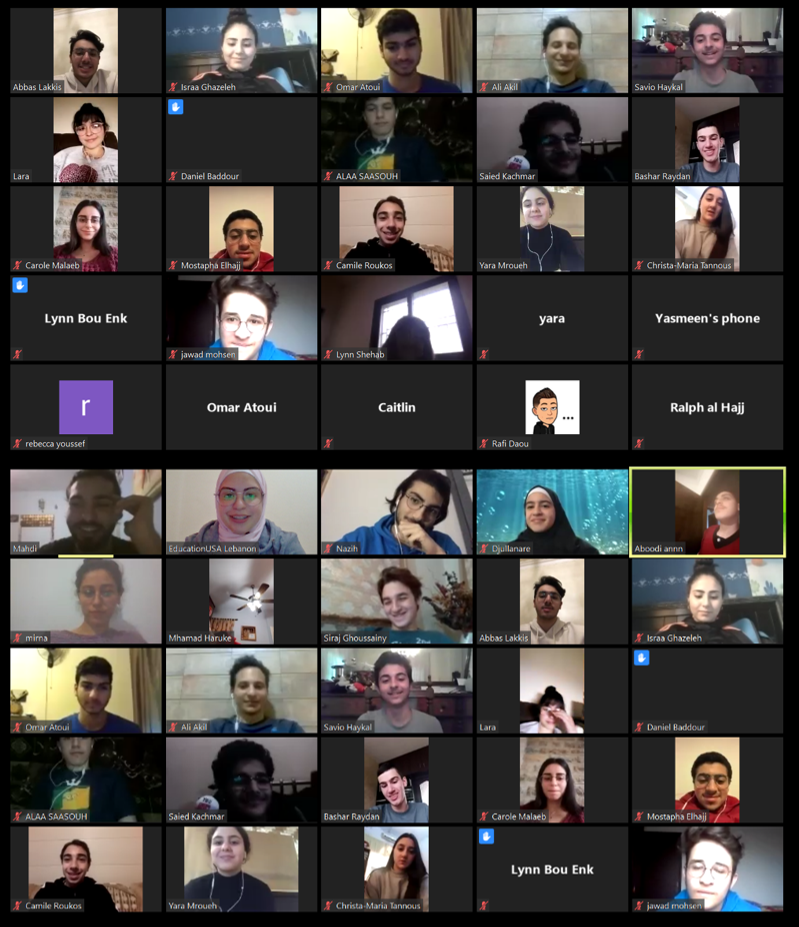Detailed description: 

The image depicts a large online video conference, possibly on Zoom. The screen is divided into a grid of 50 participants, arranged in rows of five, spanning across ten rows. Most participants have their cameras turned on, while a few have their cameras off, denoted by either initials or profile pictures.

In the center, a participant named Rebecca is represented by an 'R' in a purple box, indicating her camera is off. Nearby, other participants with their cameras off include Lynn Boenk, whose name also appears, and David Hartmore. Omar Atoui, Caitlyn, and Ralph Ataye have their cameras on, along with a participant named Rafi, who uses a cartoon image as their profile picture. 

The attendees seem to have diverse backgrounds, predominantly featuring Asian individuals, with a mix of males and females. Specifically noticeable is a participant named Mohamed Heerli, whose camera points upward, capturing his fan and light fixture instead of his face, perhaps intentionally.

Although some participants’ cameras are off or show unusual angles, most appear to be actively engaged in the video call. The image lacks visible controls or additional software interfaces, making the exact platform uncertain. 

Overall, the image gives an impression of a bustling, large-scale online meeting or conference call.